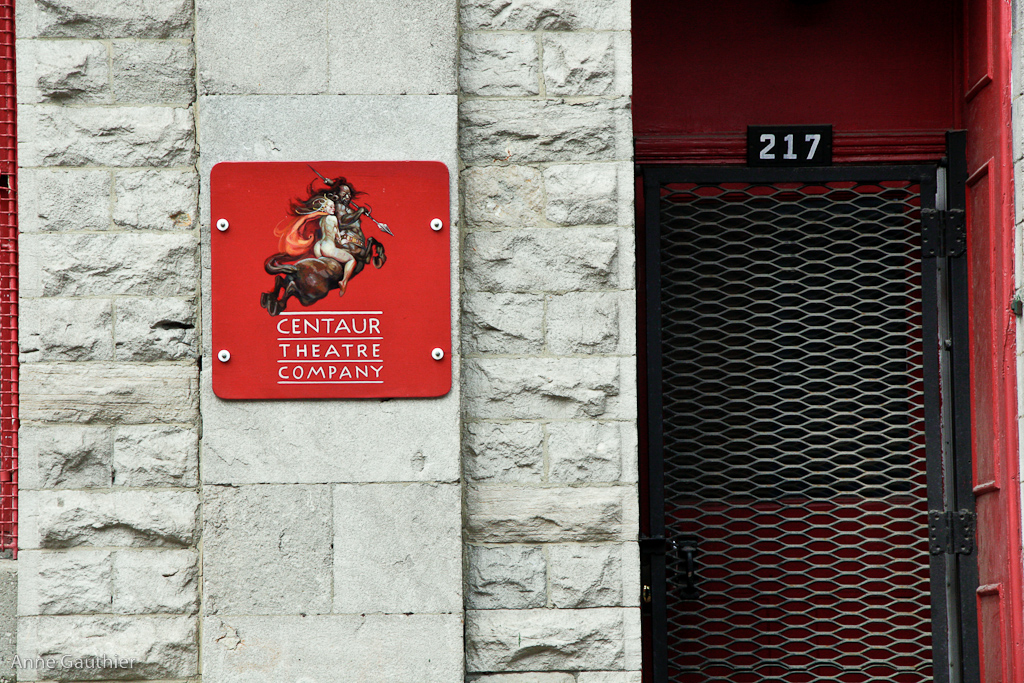The image depicts the façade of the Centaur Theater Company, characterized by a distinctive blend of rough-hewn and smoother white stone. A striking red plaque affixed with four bolts stands out against the smooth stone, featuring the company’s name and an image of a centaur holding a spear, with a naked woman donning a red scarf riding on its back. To the right of the plaque, the entrance to the theater is marked by a red-painted door framed by a black mesh screen door with a hexagon pattern. Above the door, the building number "217" is prominently displayed, guiding visitors to the theater.